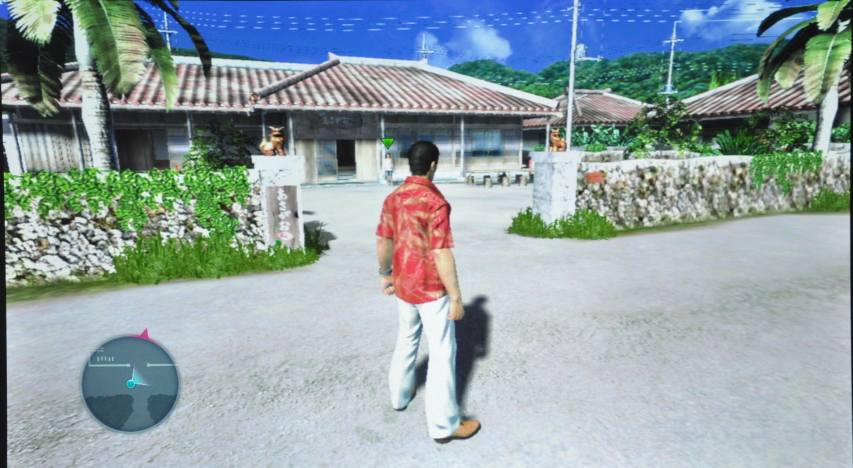This image is a detailed screenshot from a relatively recent open-world video game, reminiscent of Grand Theft Auto 5. The setting appears to be a tropical resort, potentially inspired by Hawaii, featuring lush vegetation, palm trees, and multiple island-style buildings. These buildings showcase flat-ish roofs constructed from linear logs or variegated clay tiles. 

In the background, there's a bright blue sky accented by some clouds and telephone pole power lines. The architecture includes detailed elements such as stone or brick walls with vegetation, columns flanking a driveway, and possible Japanese signage coupled with bronze sculptures, possibly deities or dogs.

In the foreground, the main character, viewed from behind, stands centrally on a gravel driveway, in front of a sprawling house. This male character has light brown skin, black hair, and is dressed in a red t-shirt adorned with orange palm tree leaf patterns, white pants, and brown shoes with a black sole. His fists are clenched, suggesting tension or readiness for action. Additionally, a green triangle above another person's head in the distance indicates they might be a target or interactive NPC. 

On the bottom left of the screen, there is a circular navigation menu, a typical in-game feature showing the character’s current location. This realistic yet somewhat graphically imperfect image typifies the immersive experience of modern sandbox adventure games.